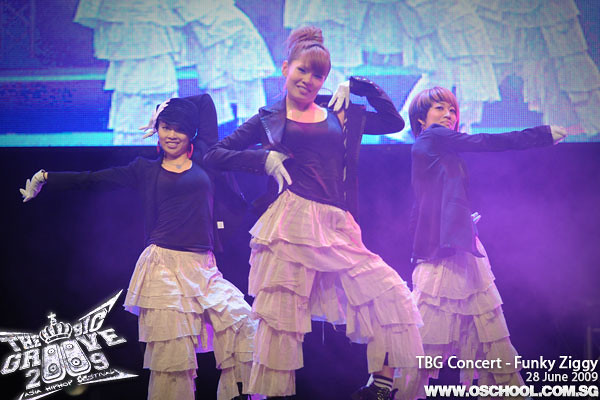The image depicts a close-up of three young Asian women on stage, likely at a concert, all striking a choreographed pose. They are dressed uniformly in black tank tops and black jackets, paired with white pants that are billowy and resemble dresses. Each woman has her hair either styled up or kept very short. The stage is bathed in blue light, emphasizing their coordinated attire. Behind them, a large projector screen displays an expanded view of their performance from a similar angle. In the lower right corner of the image, white text reads: "TBG Concert - Funky Ziggy, 28 June 2009", with a URL "www.oschool.com.sg". The lower left corner features the event's logo, "The Big Groove 2009", rendered in stylized silver text with X and crown motifs, and incorporating amplifier-like O’s.